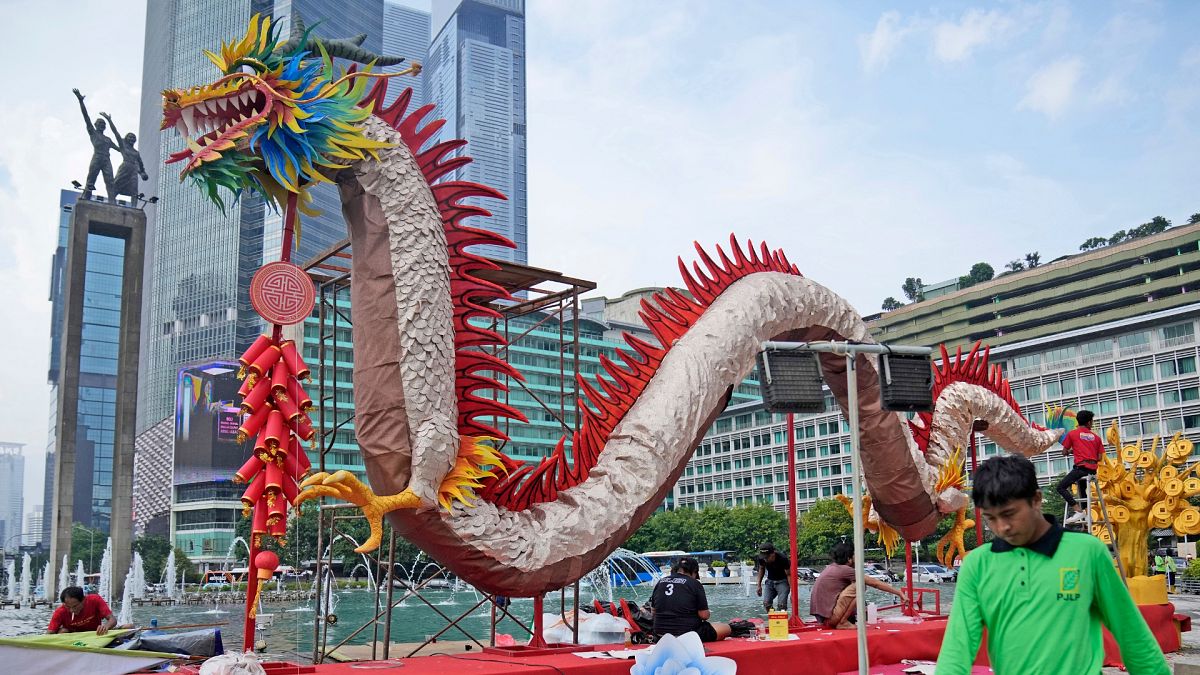This landscape photograph showcases a vibrant and intricately crafted holiday dragon float, seemingly for a Chinese New Year celebration. The dragon, depicted with meticulous detail, stretches dramatically from the top left to the bottom right of the image, its body undulating in classic serpentine curves. Its head is an arresting combination of colors: a bright red gaping mouth adorned with sharp white teeth, a blue-green-yellow gradient beard, and a dramatic cartoony white eye. Red flame-like spikes adorn its back while yellow claws reminiscent of chicken talons extend from its feet.

The background is a cityscape characterized by light blues, grays, and whites, featuring tall buildings and painted clouds in a light blue sky. One building towers on the left while an eight-story structure stands on the right. Amid this urban backdrop, a stage and distant statue add layers of depth and context to the scene. In the bottom right-hand corner, a dark-skinned man with fluffy black hair and a downward gaze is prominent. He wears a bright green shirt with a black collar and buttons, which has a yellow-outlined green leaf and letters that might spell "P-J-L-P" or "P-U-L-P" on the right side of the chest. The dragon is supported by silver poles, highlighting the technical craftsmanship behind this striking paper mâché or paper craft creation.